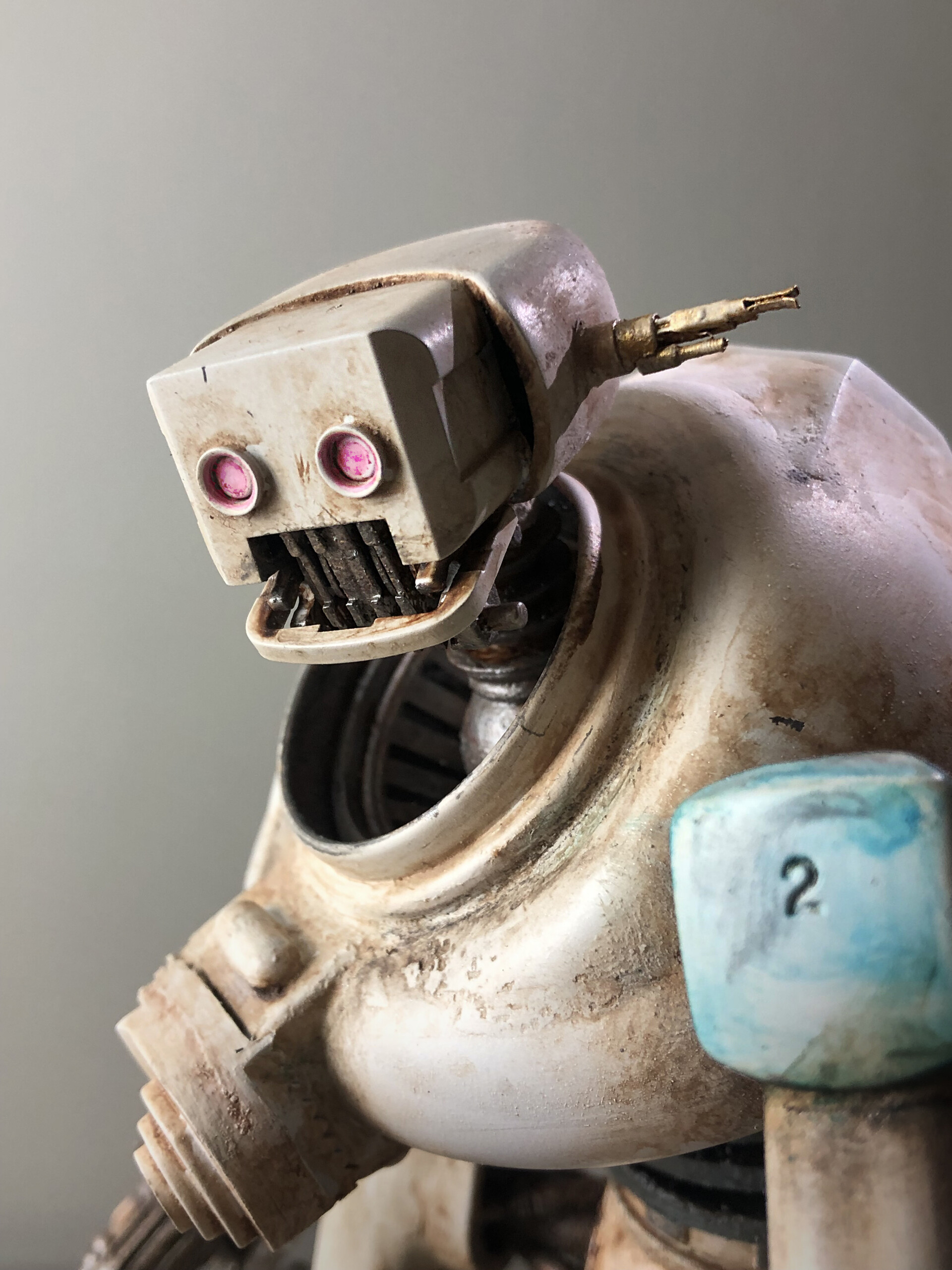The image is a tall, rectangular photograph set against a gray background, featuring a detailed depiction of a robotic figure. The robot itself appears quite distinctive and somewhat menacing, almost as if it could be a villain in a movie. The head of the robot is square, crafted from a pinkish-beige metal that looks dirty and rusted, with a metallic piece protruding from the side and something sharp sticking out of the back. Its eyes are round, colored in with what looks like pink marker, reflecting a crude, hand-drawn quality. The mouth area resembles black piano keys, with a metal piece extending from what would be its lower lip, adding to its grim appearance.

Beneath the head, the neck is skinny and the neck hole is notably wide, with a big, silver pewter-colored metal protruding down. The main body of the robot resembles a flower pot, crafted from the same dirty, pinky silvery metal as the head. On the right side of the torso, there is a conspicuous blue and white square object featuring a bold number 2, similar to a large marshmallow in shape, which stands out as the lightest colored element in the image. The right arm of the robot, which gets thinner toward what would be the forearm, extends out but is cut off at the waist, leaving the lower part of the robot unseen. The entire robot's design exudes a sense of dirtiness and griminess, with various shapes jutting out, contributing to its overall sinister and fantastical appearance.